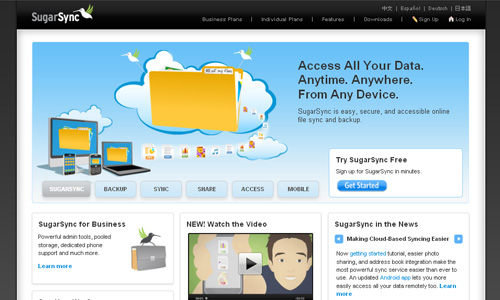At the top left corner, the image features the logo and name "SugarSync" accompanied by a graphic of a bird. Below it, navigation options are listed: Business Plans, Industrial Plans, Features, Downloads, Sign Up, and Log In. Language options are displayed above these: Japanese, Español, Dutch, and Korean.

The main portion of the image showcases a large visual centered around the tagline: "Access all your data anytime, anywhere, from any device." This is followed by a description: "SugarSync is easy, secure, and accessible online via a sync backup." The background contains icons of folders and clouds, alongside illustrations of a monitor, laptop, and smartphone.

Further down, key service features are highlighted in sequential blue boxes: Backup, Sync, Share, Access Mobile. A call-to-action invites users to "Try SugarSync first" and "Sign Up for SugarSync in minutes," with a blue button labeled "Get Started."

The business section is detailed under "SugarSync for Business," focusing on powerful admin tools, ample storage pools, dedicated phone support, and more. An icon of a suitcase represents this section. Below, there's an option to "Watch the Video," which shows someone using a smartphone with accompanying cartoon illustrations.

Towards the end, "SugarSync in the News" features highlights about making cloud-based syncing easier, accompanied by a "Getting Started Tutorial" and "Photo Sharing Address" to wrap up the visual contents.